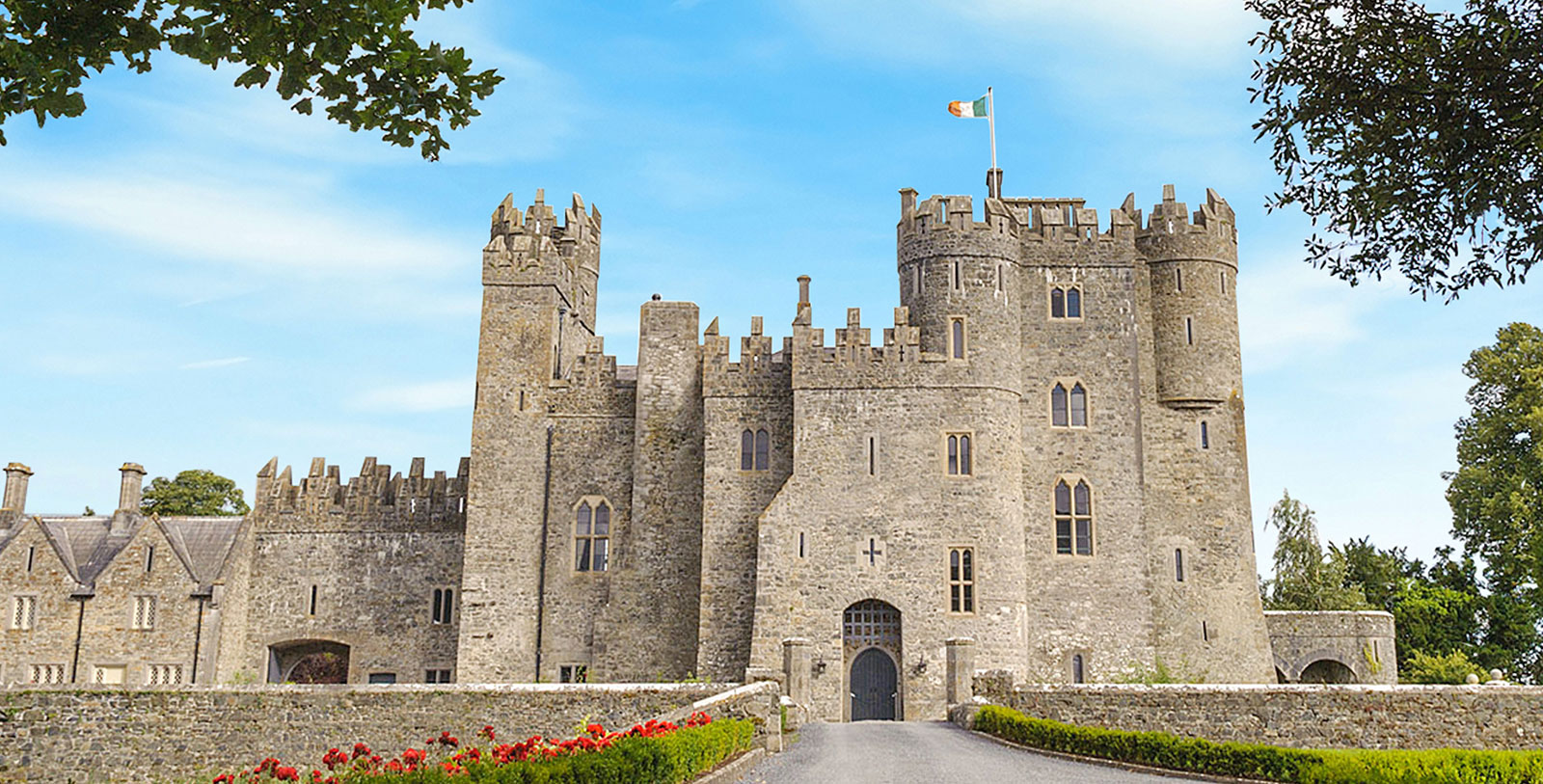The image depicts a meticulously maintained French castle estate on a bright spring or summer day. The horizontally framed photograph captures the castle's imposing gray stone structure under a vibrant blue sky, adorned with a few wispy white clouds. The central focus is the largest section of the castle standing about four stories tall, with a shorter two-story extension on the left. This main part features an arched front door and narrow vertical windows, with a few rounded turrets that subtly extend above the main building. At the very top, a flagpole hoists a tricolor flag with vertical green, white, and orange stripes.

In the foreground, overhanging tree branches and foliage frame the scene, while behind the castle and along the sides, trees with lush green leaves add to the picturesque setting. The entryway or driveway leading up to the castle is bordered by neatly trimmed shrubs and blooming red tulips, enhancing the estate's charm. A light gray stone fence encircles the property, contributing to its overall grandeur. The paved walkway leading to the front entrance further emphasizes the castle's well-kept and beautifully maintained appearance.